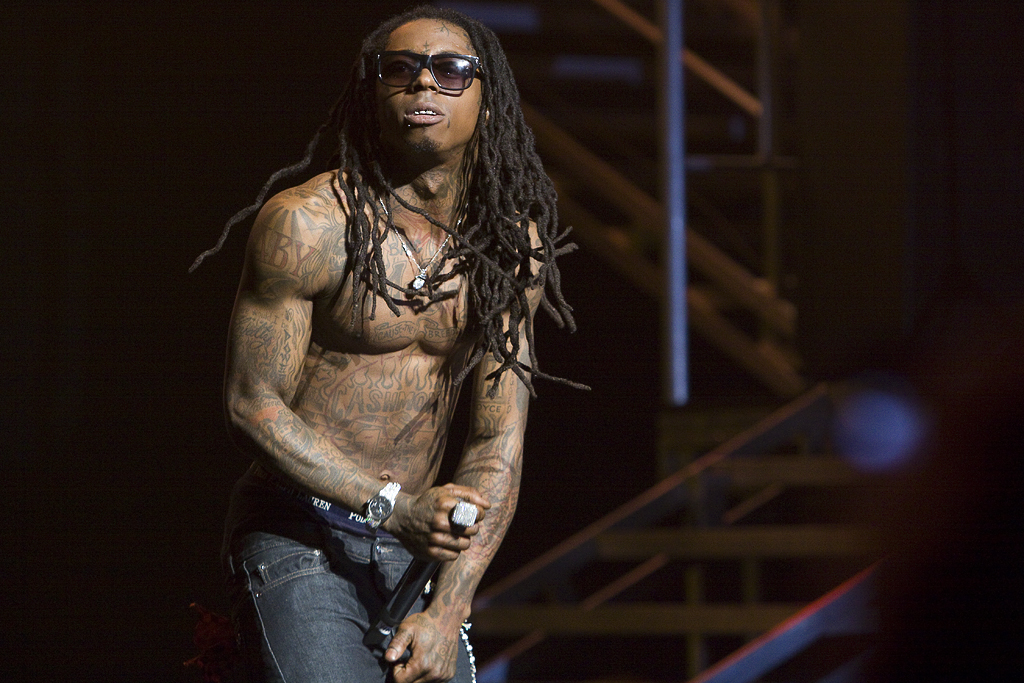In this image, an African-American rapper, who might be Lil Wayne, is captured mid-performance. The rapper, positioned slightly left of center, stands on stage, sporting large, long dreadlocks cascading over his shoulders, and stylish black sunglasses. His face is clean-shaven and his mouth slightly open, revealing his teeth as if he's mid-rap. His entire arms, chest, and neck are adorned with a multitude of tattoos, emphasizing his muscular physique, as he is shirtless. 

He wears a prominent silver watch on his right wrist, complemented by a large silver ring on the pointer finger of the same hand, which also firmly grips a microphone. His left arm hangs down by his side. Below, he is dressed in dark blue jeans, with the waistband of his dark blue Ralph Lauren underwear peeking out, marked with white lettering. 

The background is somewhat dim and blurry, featuring a brownish-gray hue, with elements that resemble a metal staircase or railing, contributing to the industrial, stage-like setting where the performance is occurring.